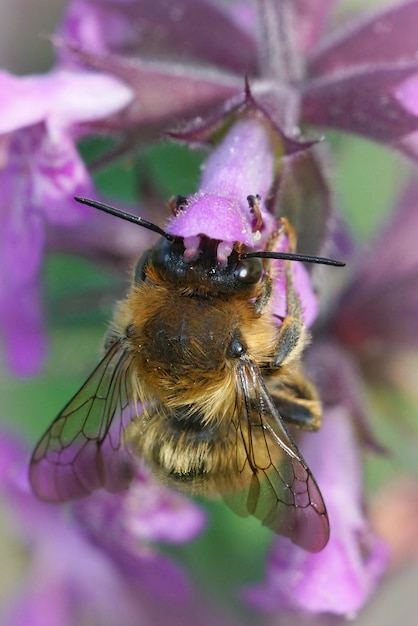This highly detailed daylight photograph captures a close-up view of a bee clinging to a vibrant purple flower outdoors. From above, we see the bee's back with its head partially inside the flower, its black eyes peeking out from the sides, and its antennae protruding outward. The yellow and black-striped bee, covered in tiny hair-like bristles, latches onto the flower with its legs wrapped securely around the petals. Its transparent wings, interlaced with fine black lines, are spread outward, revealing the intricate details of its structure. The purple flower, characterized by long, cup-shaped petals, surrounds the central scene, with more of the flower visible but blurred in the background. This soft, out-of-focus backdrop highlights the sharpness and clarity of the bee, accentuating its pollen-dusted lower legs and body. The detailed, high-resolution image offers a striking and intimate glimpse into the bee's world as it interacts with the flower.